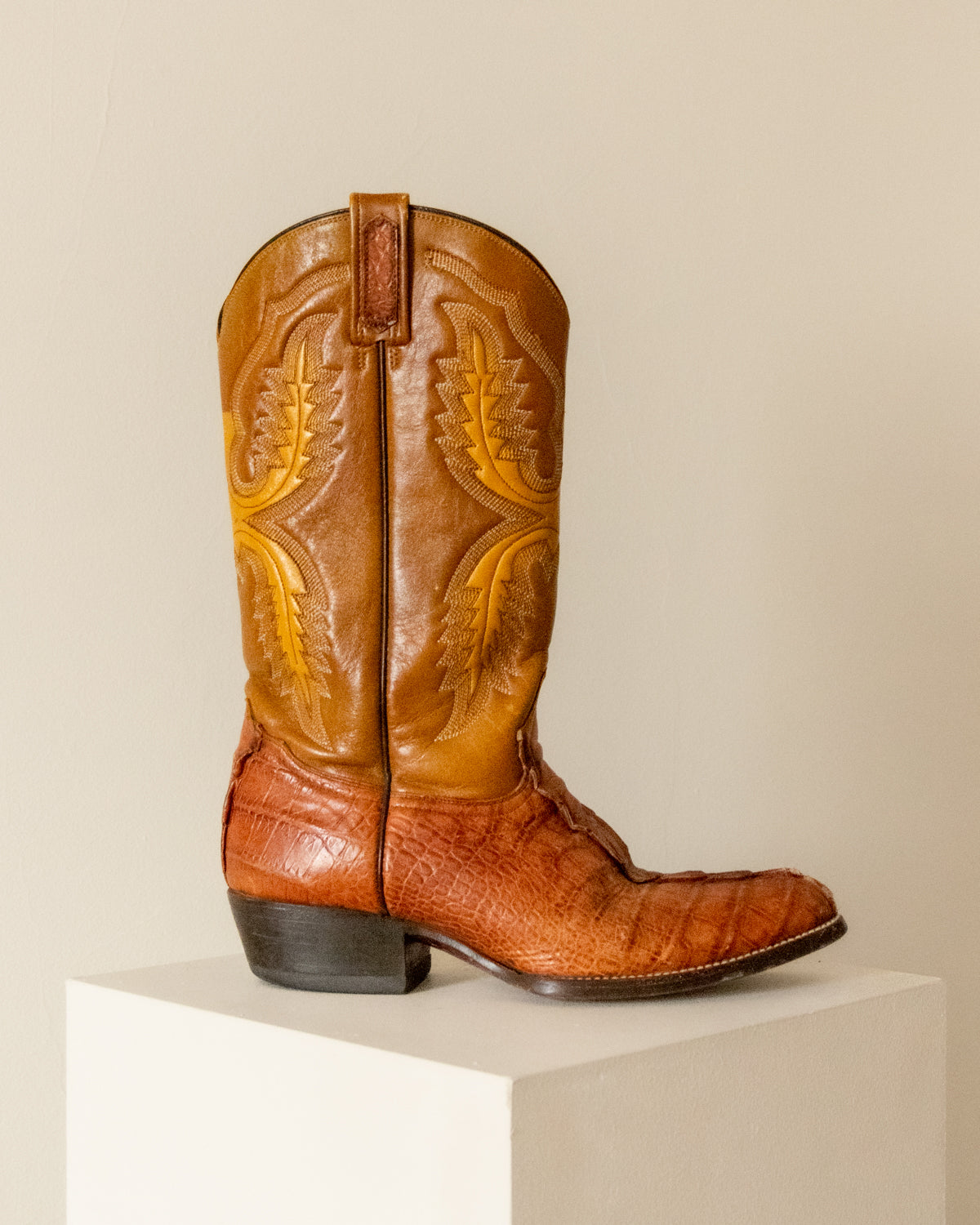The image depicts a carefully arranged display of a single cowboy boot, positioned on a white, cube-like pedestal. The background is a subtle gray to off-white, ensuring minimal distraction from the boot. The boot, designed with a dark brown heel and sole, showcases leather transitioning from a rusty orange at the base to a lighter tan brown towards the top. Intricate patterns resembling leaf designs or zigzag embroidery in a yellowish-brown hue adorn the upper part of the boot. The leather at the bottom sections of the boot suggests a texture similar to snakeskin or alligator skin. The boot is approximately knee-high, with a low heel, and is viewed from the side with the toe pointing to the right. The overall aesthetic implies a setting akin to an art gallery, emphasizing the boot as a noteworthy piece, possibly dating back to the 1960s or 1970s.